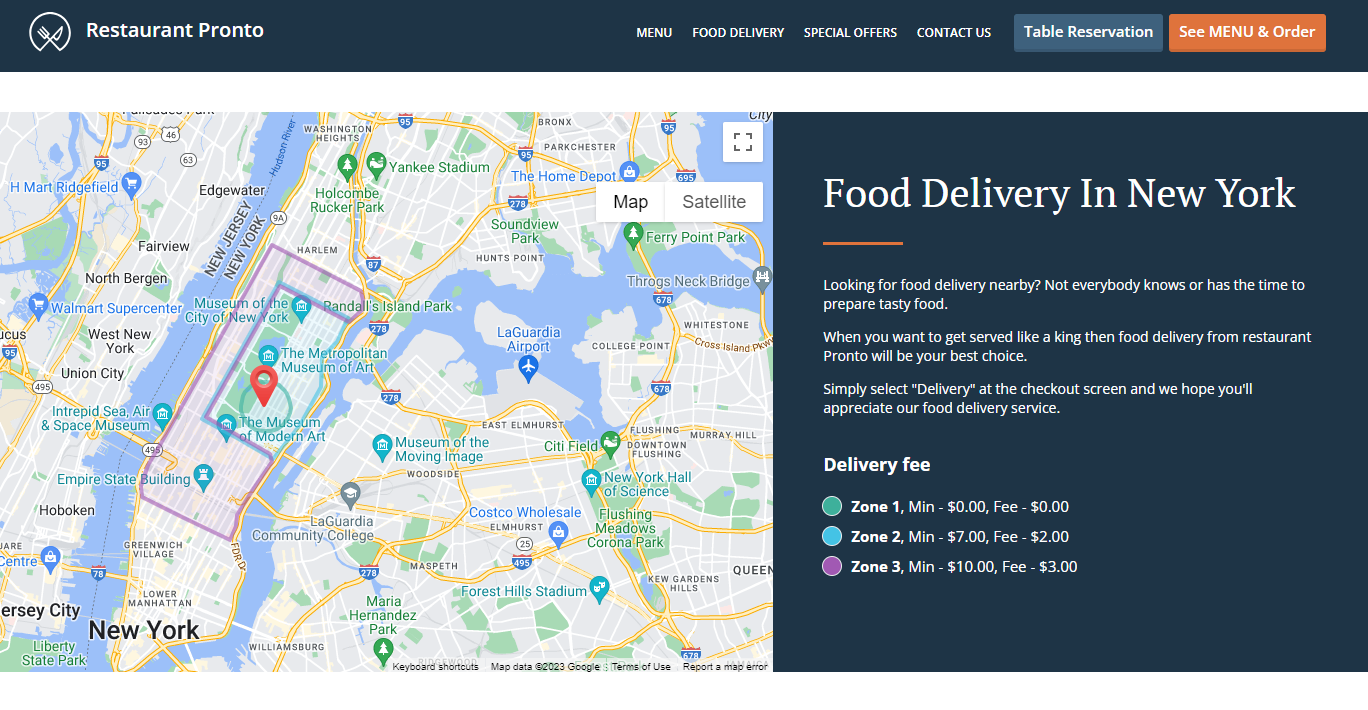A widescreen landscape screenshot captures the homepage of the Restaurant Pronto website, as viewed on a desktop or laptop computer. At the top of the page, a dark green banner prominently displays the restaurant's name, “Restaurant Pronto,” accompanied by the establishment's icon – a semicircle formed by a crossed fork and knife. 

To the right of the banner, there are a series of navigation buttons: "Menu," "Food Delivery," "Special Offers," "Contact Us," followed by "Table Reservation" (highlighted with a light blue background) and "See Menu and Order" (highlighted in orange).

Immediately below the banner, a Google Maps interface showcases the restaurant's location in the heart of Manhattan, New York. The map also marks various other locations spread across New York and New Jersey.

On the right side of the screen, an informational box details the restaurant's food delivery service. The text reads: 

"Food delivery in New York. Looking for food delivery nearby? Not everybody knows or has the time to prepare tasty food. When you want to get served like a king, food delivery from Restaurant Pronto will be your best choice. Simply select delivery at the checkout screen, and we hope you'll appreciate our food delivery service."

The delivery fee section outlines the costs for different zones:
- Zone 1: No fee
- Zone 2: $7.00
- Zone 3: $10.00 

This well-organized homepage gives a clear overview of Restaurant Pronto’s offerings and their convenient location in New York.